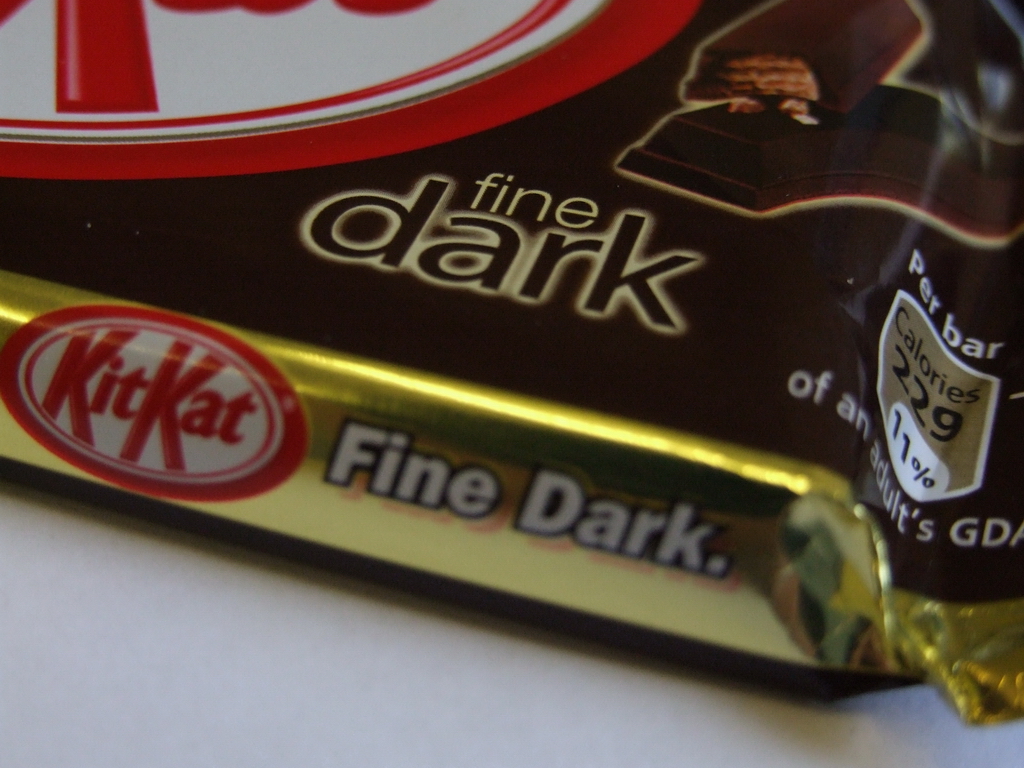This close-up image showcases the corner of a KidKat chocolate bar wrapped in a sophisticated foil material. The wrapper features a rich color scheme with a dark brown top and golden sides, complemented by a striking red and white label. Despite its partial view, the packaging remains sealed, indicating that the chocolate bar is unopened. The wrapper boldly announces "Fine Dark" chocolate and specifies its calorie content as 229 per bar. In the top right-hand corner, a small image depicts the chocolate bar itself: a thin, dark brown exterior with a broken piece revealing a lighter brown interior. The detailed design and enticing visuals make it clear that this is a premium dark chocolate treat.